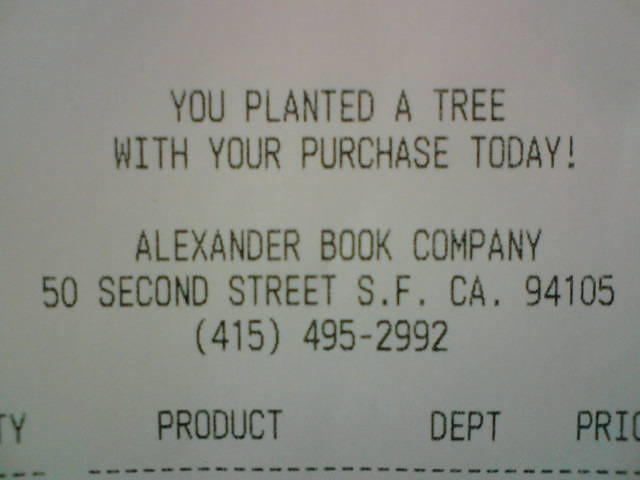A detailed close-up photograph captures a portion of a receipt, which likely started out as white but now appears to have a grayish-lilac tint. The receipt is oriented horizontally and is rectangular in shape. The top section of the receipt features bold, capital letters that read: "YOU PLANTED A TREE." Directly below, it continues with another line in capital letters: "WITH YOUR PURCHASE TODAY!" 

Further down, separated by a couple of blank lines, the text reads: "ALEXANDER BOOK COMPANY," also in all capital letters. The next line provides an address: "52ND STREET, S.F.CA.94105," with the ZIP code, "94105," repeated for emphasis.

Two lines below is a partially obscured word, followed by the word "PRODUCT." This is followed by the abbreviation "D.E.P.T," another space, and the partially visible text "P.R.I," likely short for "PRICE." Below this section, a dotted black line runs horizontally across the width of the receipt.